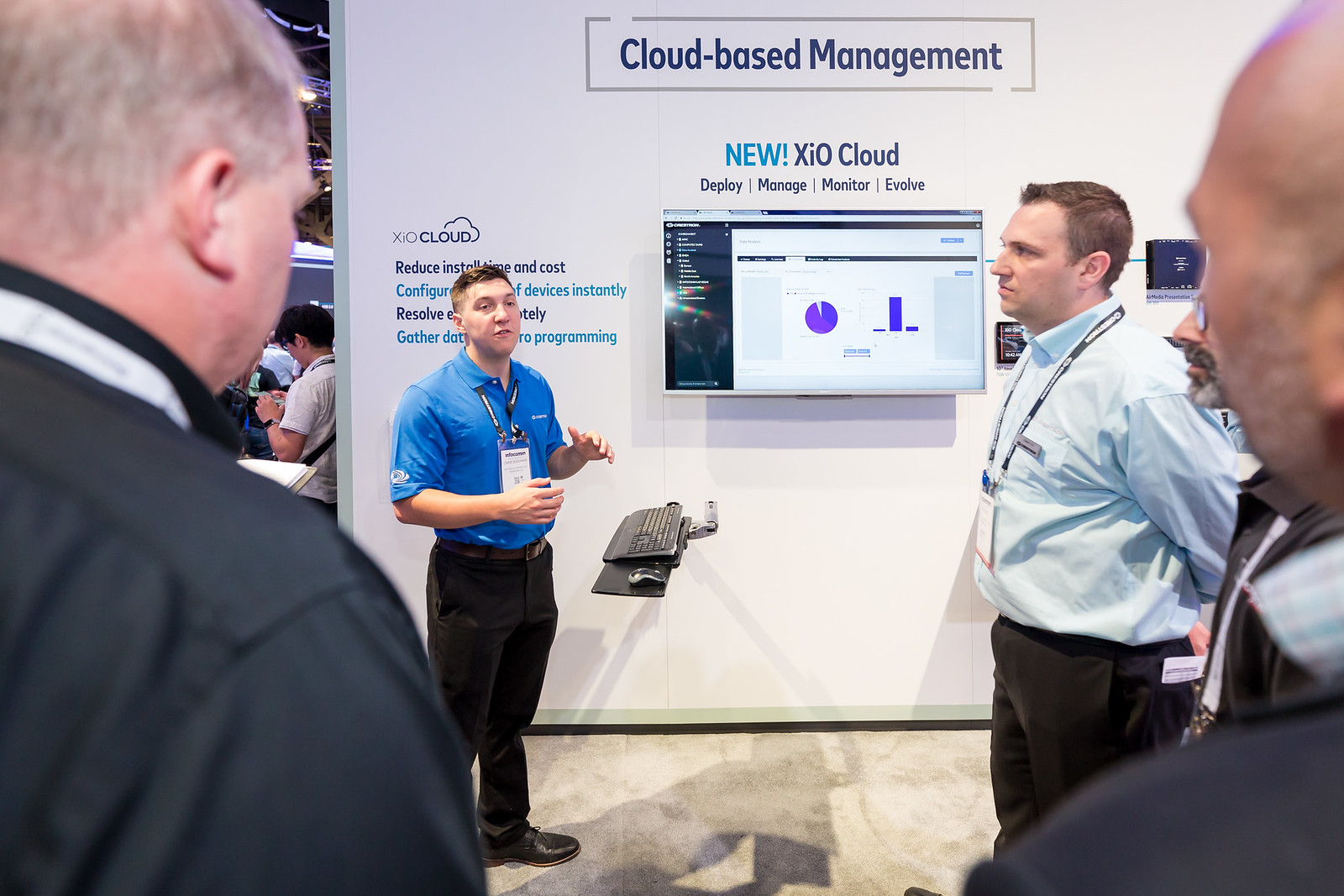The image depicts a scene from an I.T. show featuring a presentation on "Cloud-Based Management" and the "new X.I.O. Cloud." The text on the white wall behind the speaker includes phrases like "Deploy, Manage, Monitor, Evolve," although some text is obscured. Central to the scene is a man in a blue button-up shirt with rolled-back sleeves, black pants, and a lanyard badge. He is animatedly gesturing and mid-speech, standing in front of a computer monitor mounted on the wall, connected to a platform with a keyboard and mouse. To his right is another man in a light blue button-up shirt tucked into black slacks, also wearing a lanyard badge but remaining silent and facing left. Observing the scene are two men in black shirts and several other individuals dressed in office attire, consisting of lightweight jackets and button-down shirts. The atmosphere is focused and professional, with attention centered on the speaker and the digital display.